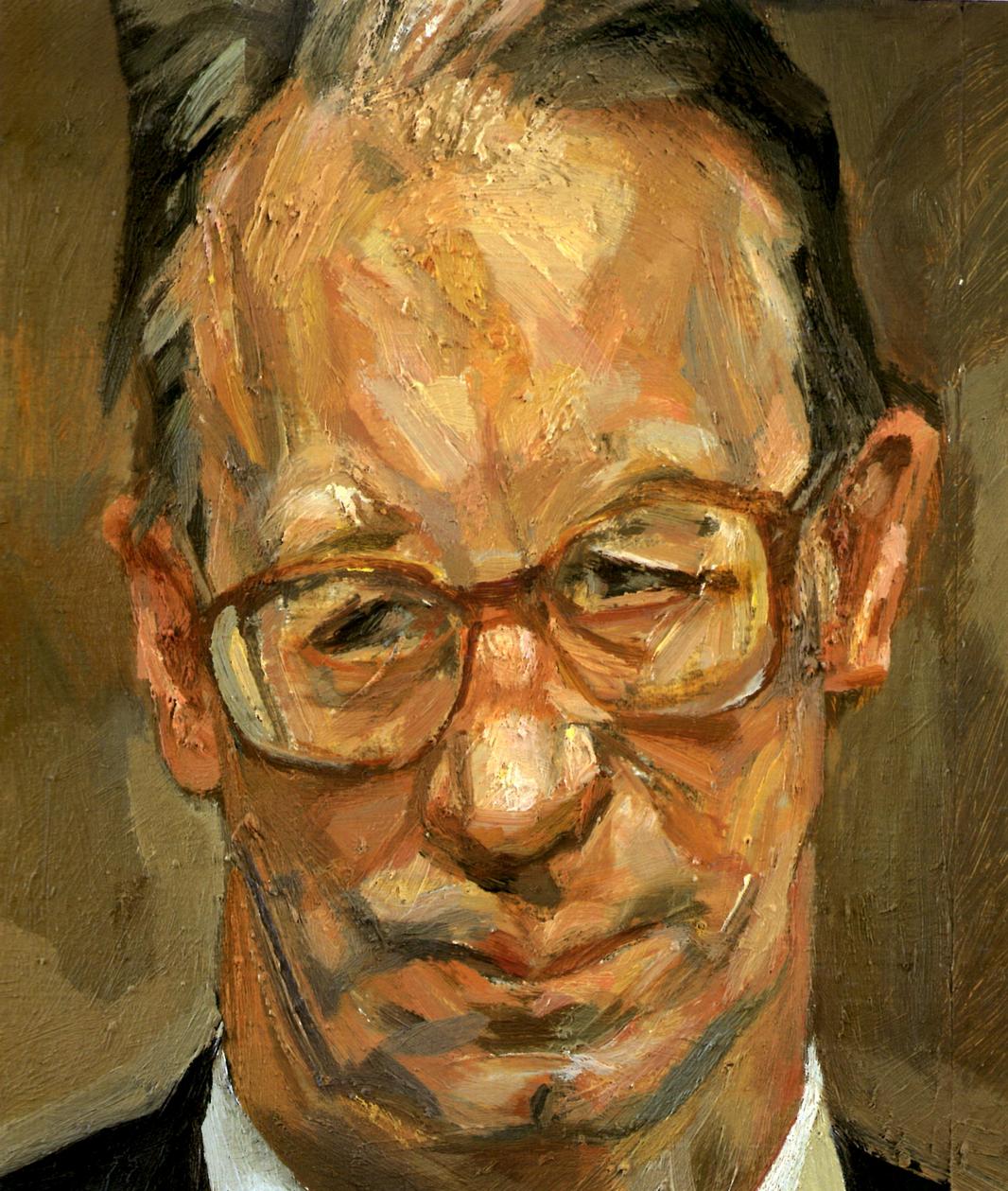The image depicts an oil-based painting of an older man, likely aged between 60 and 70, with a dignified and stern expression on his face. His face is the main focus, occupying the majority of the frame, from the base of his neck and shoulders upwards. The man has a light skin complexion with shades of pink and some gray toning under his chin. He wears brown-framed glasses, and his hair is predominantly dark brown with gray streaks, especially prominent along the middle and sides. He is dressed in a white shirt with a typical collar, complemented by a black suit coat or tuxedo. The background of the painting features warm yellow and brown tones, adding a touch of depth and age to the portrait. The detail in the man's facial features and attire suggests that this is a meticulously crafted and well-executed painting, possibly of a recognizable 20th-century figure. The overall setting is clear and devoid of any signatures, words, or numbers.